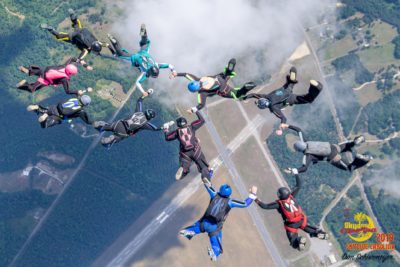The image depicts a group of approximately 14 skydivers captured from a high-altitude, overhead perspective. Despite the low quality, the figures are clearly seen in the formation of a large circle, holding hands as they descend through the sky. Each skydiver is equipped with a helmet and wears a distinct body suit in colors ranging from blue, black, and teal to pink, red, and gray. Backpacks in various shades such as red and pink are visible, likely containing their parachutes which have not yet been deployed. Below them, the distant ground presents a patchwork of green trees, grass, and brown fields. A notable feature of the landscape is a crossing of two roads, creating an X-shaped intersection, alongside wispy white clouds at the top center of the image, partially obscuring the view below.